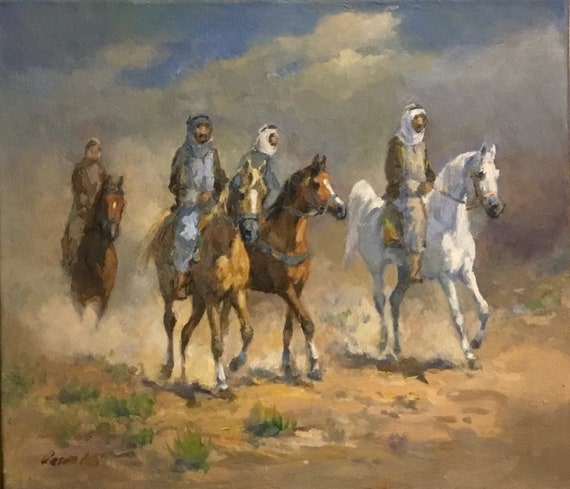In this evocative watercolor painting, four Arabic men are seen galloping across a desert landscape on horseback. The men are clad in long dress-like fabrics with coats draped over them, their heads wrapped in scarves secured with cords, shielding their faces from the elements. The scene captures the dynamic motion of the horses: a striking all-white Arabic horse with an upright tail is ridden by a man in a beige outfit and white head covering, while the other three horses, in varying shades of brown with white markings on their noses, are ridden by men in blue and white coverings. A substantial cloud of dust is churned up behind them, hinting at the windy conditions. The ground beneath them is a brown, sandy expanse, blending seamlessly into the dust and clouds billowing in the background. Above, blue skies and sunlight permeate the scene, casting light over the figures and animals, enhancing the painting's impressionistic quality. At the bottom left of the artwork, a barely legible artist’s signature and some sparse vegetation can be discerned, adding to the painting’s subtle details.